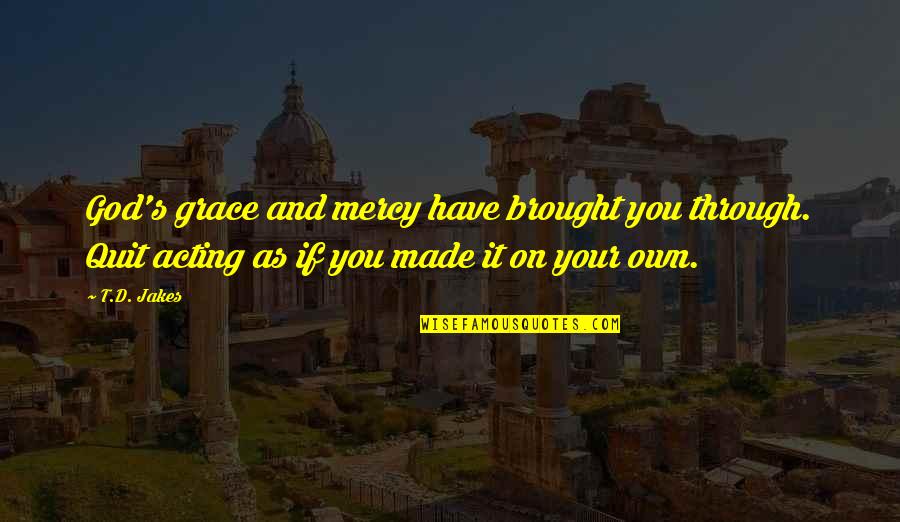The image features a darkened, almost transparent photograph of the Roman Forum in Italy, characterized by its ancient, crumbling columns and stone structures surrounded by patches of green grass. The faded grandeur of the ancient site is visible despite the dimness. Overlaid on this historic backdrop, a poignant quote in bright yellow cursive font reads: "God's grace and mercy have brought you through; quit acting as if you made it on your own." This inspirational message, attributed to T.D. Jakes, includes a reference to wisefamousquotes.com in bold black text with a yellow background, subtly placed below the quote.